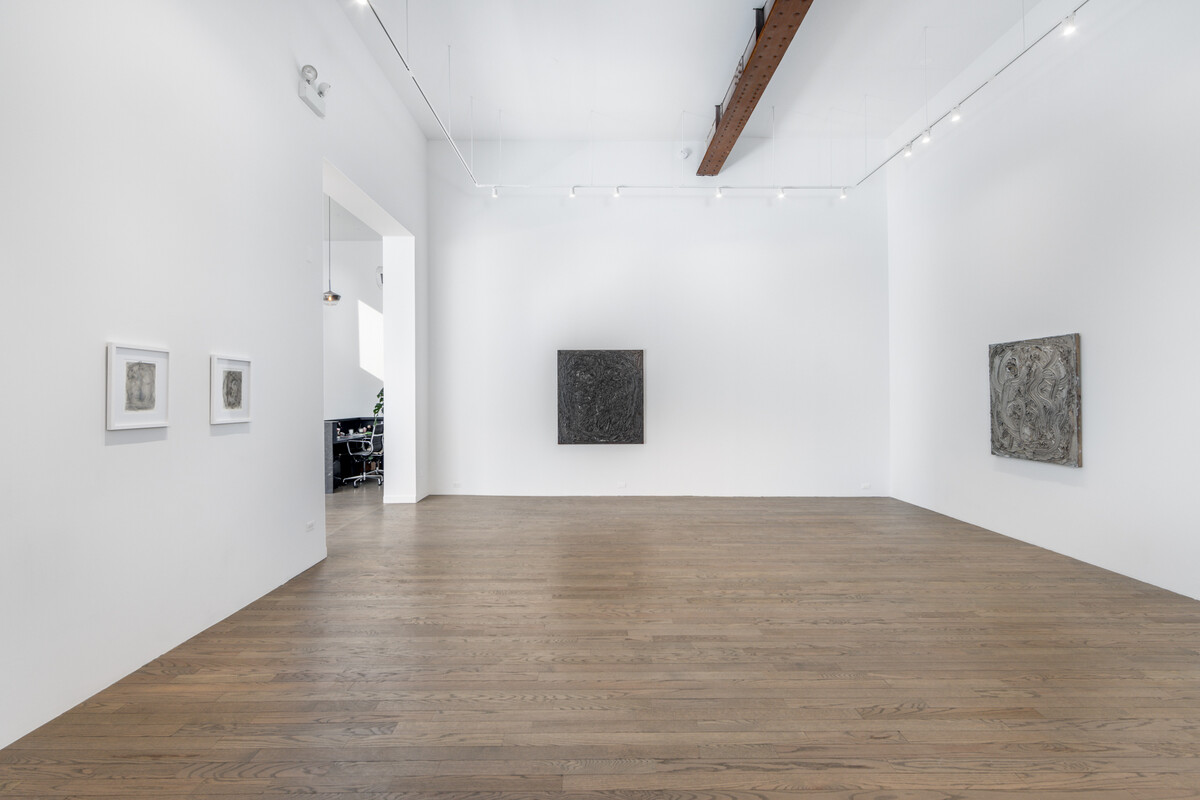The well-lit and meticulously arranged art gallery showcases an elegant and minimalist design, featuring stark white walls and oak-colored hardwood flooring. The flat white ceiling is adorned with a perimeter of track lighting and a lighting strip, ensuring optimal illumination. On the wall to the left, two smaller, white-framed prints are displayed side by side, creating a set. Directly ahead hangs a striking large black canvas adorned with intricate, swirling patterns. To the right, there is another substantial canvas with textured, silvery swirls. Prominent within the room is a metal beam with rivets, extending across the ceiling and enhancing the industrial aesthetic. Through a large entryway, topped with emergency lighting, a glimpse into another area reveals a sophisticated black desk accompanied by a sleek black and metal office chair, illuminated by hanging chandelier lights.